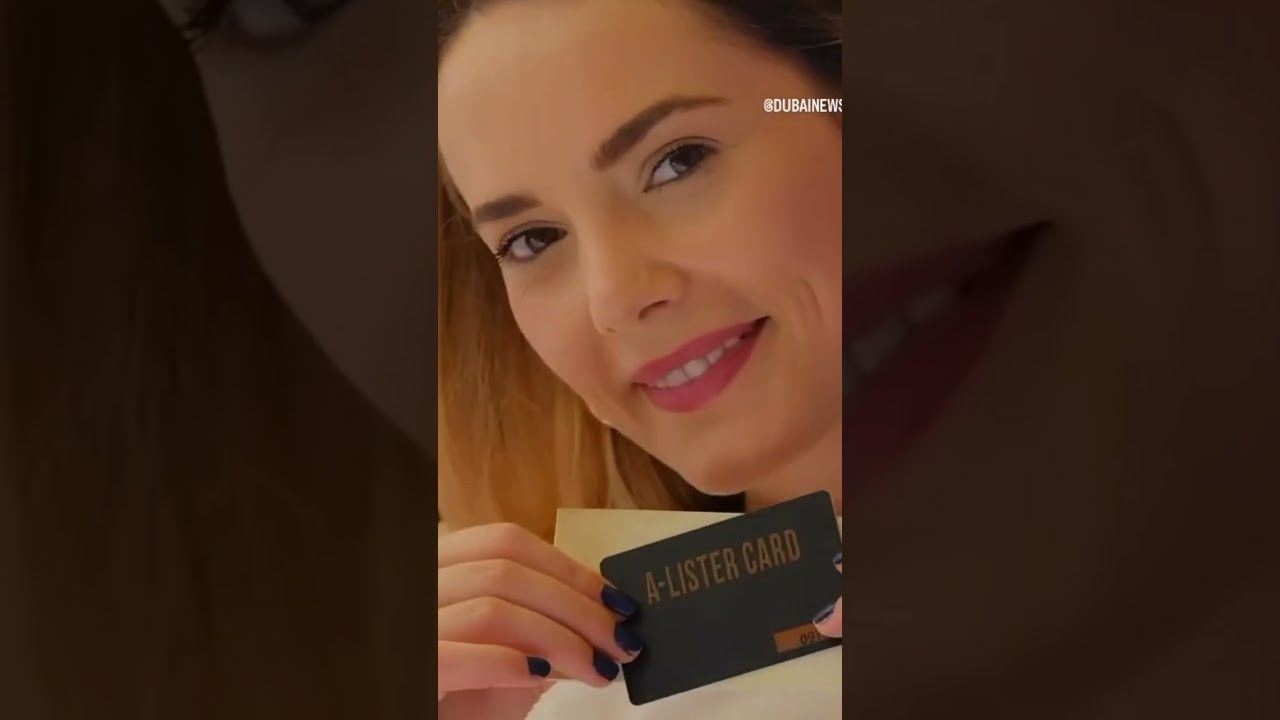The image features a woman centered in a three-panel composition. The main, brightly lit central panel captures a close-up of her face, where she smiles and tilts her head slightly to the side. She is wearing pink lipstick and sporting black nail polish. In her hand, she holds a card labeled "A-Lister Card," which is gray with a gold label. Behind this card, there seems to be another light-colored card, possibly yellowish or white. The woman's hair transitions from dark shades near the roots to light brown or almost blonde at the tips.

The left and right panels display extreme close-ups of the same central image but are heavily darkened to the point of being almost black-and-white. Despite the darkening, you can discern her lips on the right panel and part of her eye and face on the left panel. There's also some partially obscured text on the card in the upper right corner of the main image, which appears to say "At Dubai News," though part of it is cut off. She seems proud, possibly showcasing her "A-Lister Card" with confidence.